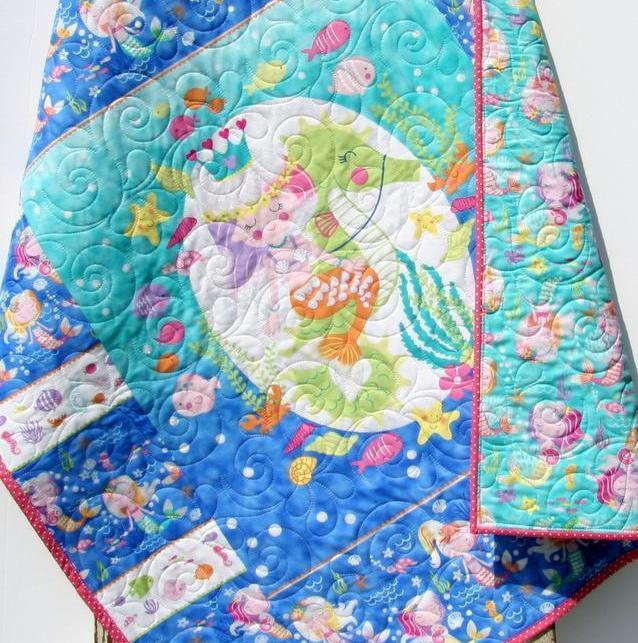This close-up image captures a square-shaped, professionally photographed quilt designed for a little girl with an under-the-sea theme. The main color palette of the quilt is blue, reflecting its oceanic theme. The center of the quilt features a large white oval, showcasing a cheerful mermaid with pink and purple hair, a blue crown adorned with pink and red hearts, and an orange tail decorated with white hearts. She is riding a cheerful green seahorse with pink cheeks. Surrounding the central oval, the blue background is filled with various sea animals and smaller mermaids swimming among bubbles. The quilt's edges feature alternating squares of fish and sea creatures, all rendered in bright, child-friendly hues like baby blues, greens, pinks, and yellows. The right side of the quilt is folded over, revealing a uniform backside with an under-the-sea pattern, consistent with the playful aquatic theme.